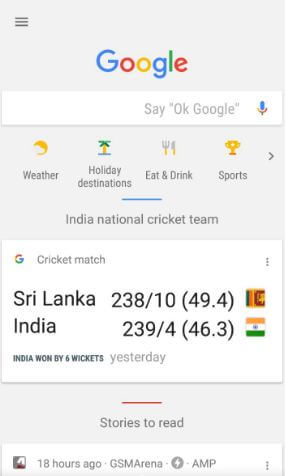Screenshot depicting a minimalist Google search interface set against a plain white background. The iconic "Google" logo is prominently displayed at the top. Directly below the logo is the prompt “Okay, Google,” followed by a series of commonly searched categories including "Weather," "Holiday Destination," "Eat & Drink," and "Sports." Each category is accompanied by a corresponding icon: a crescent moon for "Weather," a palm tree for "Holiday Destination," a fork and knife for "Eat & Drink," and a trophy for "Sports."

Underneath these categories, there is a segment on Sri Lanka, showing scores for a cricket match, followed by information regarding an India cricket match. Further down, the screen contains a section titled "Stories to Read," written in gray text. Adjacent to this section is a short horizontal red line. The final piece of text on the screenshot reads "18 hours ago," indicating the recency of the content.